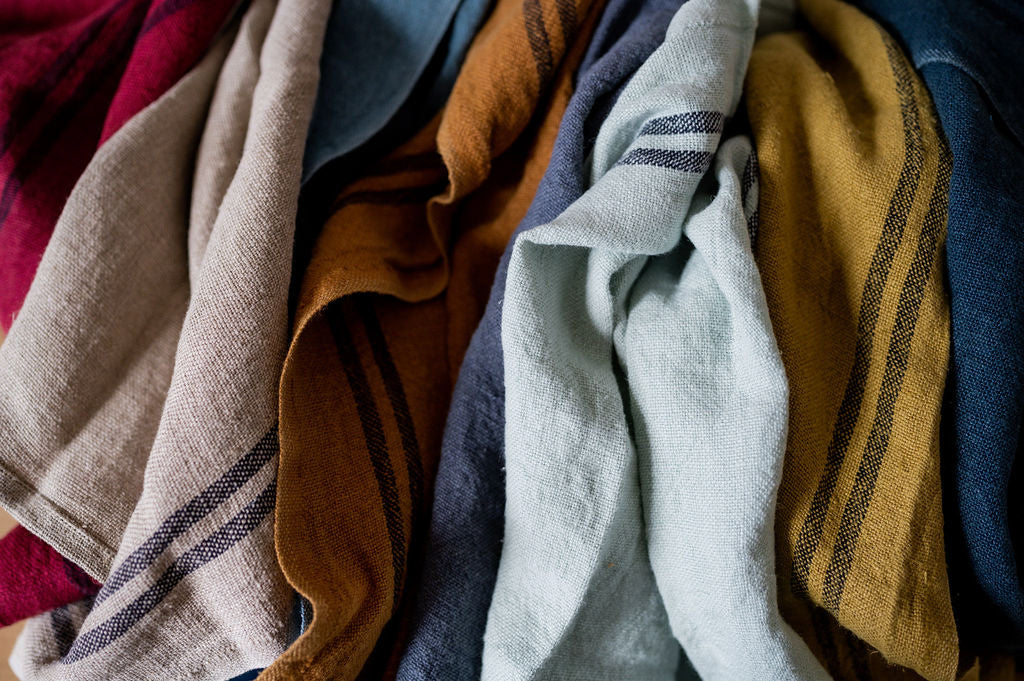The image features an assortment of variously colored thin cotton cloths, possibly towels, that are bunched together and appear to be hanging. Positioned in a semi-ordered row from top to bottom, and extending left to right, the arrangement begins with a red cloth featuring a black stripe. Slightly overlapping this, a tan cloth with two dark brown stripes is visible. Neighboring it is an orange cloth, accented similarly with two black stripes, partially covering a glimpse of a light blue cloth at the top. Adjacent to the orange cloth, a dark blue trim is visible, leading to a nearby light blue cloth distinguished by two navy blue stripes. Further right, a dark yellow cloth with two black stripes is partly obscured by another dark denim-colored cloth at the far end. Altogether, these cloths produce a visually intriguing collection of varied hues and stripe patterns.